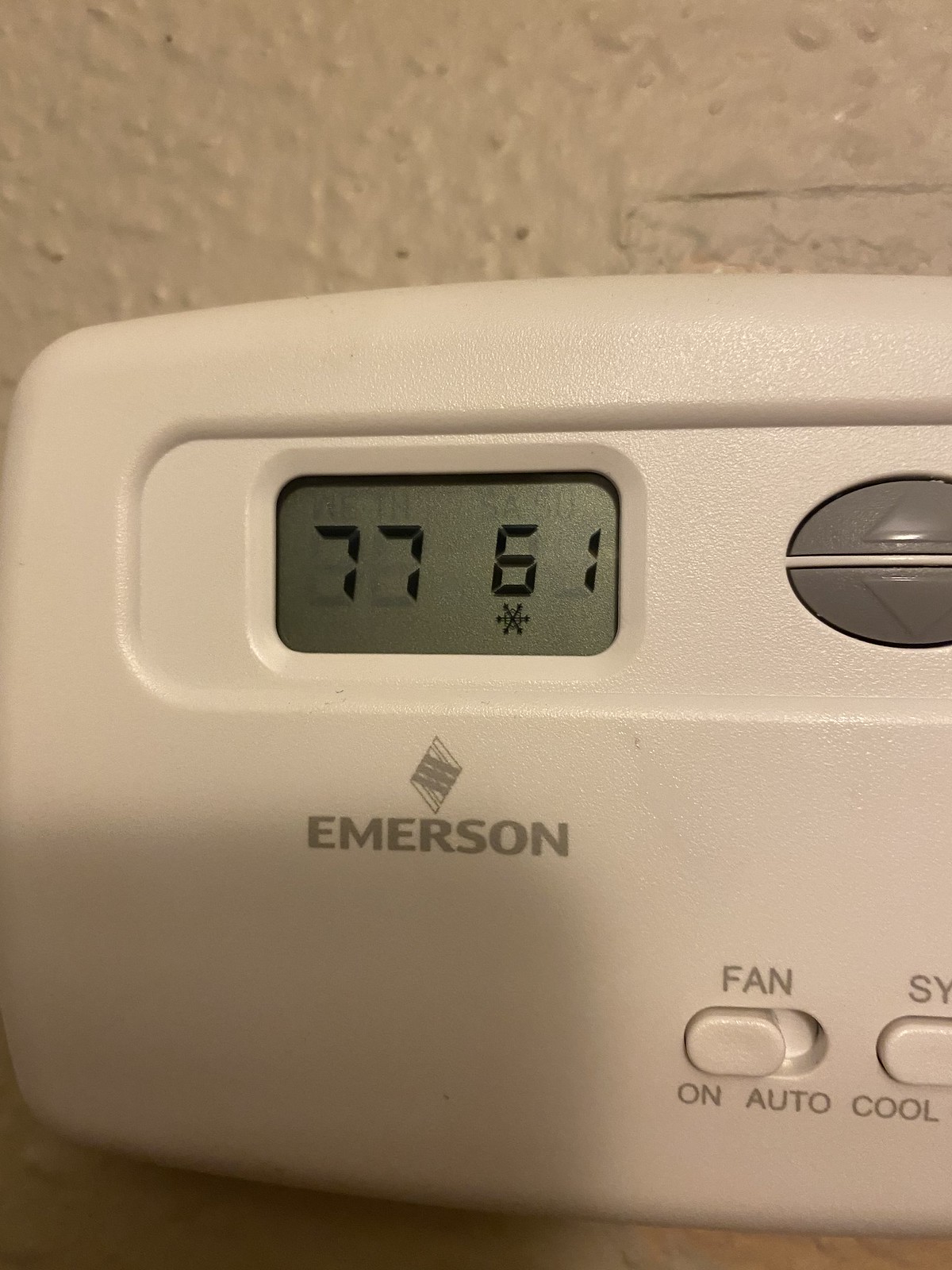This up-close photograph showcases an Emerson thermostat unit. The main body of the thermostat features a white, slightly textured surface, occupying the majority of the bottom three-quarters of the image. The visible portion of the thermostat is predominantly on the left side, as the right side is cut off from view. The background is a light gray, textured wall, providing a subtle contrast to the white thermostat unit.

In the bottom left quadrant of the image, a shadow partially obscures both the thermostat and the wall. At the center of the thermostat, slightly to the left, there is an open LCD screen displaying the numbers "77" and "61" in black computerized digits. This likely indicates the cooling range set to 67°F and heating to 61°F. Beneath the "67," there is a small six-pointed snowflake symbol in black. The LCD background appears to be a shiny gray surface.

To the right of the LCD screen, there is an oval-shaped area with two gray buttons, split horizontally by white plastic. The top button features an up arrow, while the bottom button has a down arrow. Additionally, two small white pill-shaped switches at the bottom are labeled "Fan," "On," "Auto," and "Cool," with another switch partially visible, displaying "SY." These dials can likely be slid back and forth to adjust the settings.